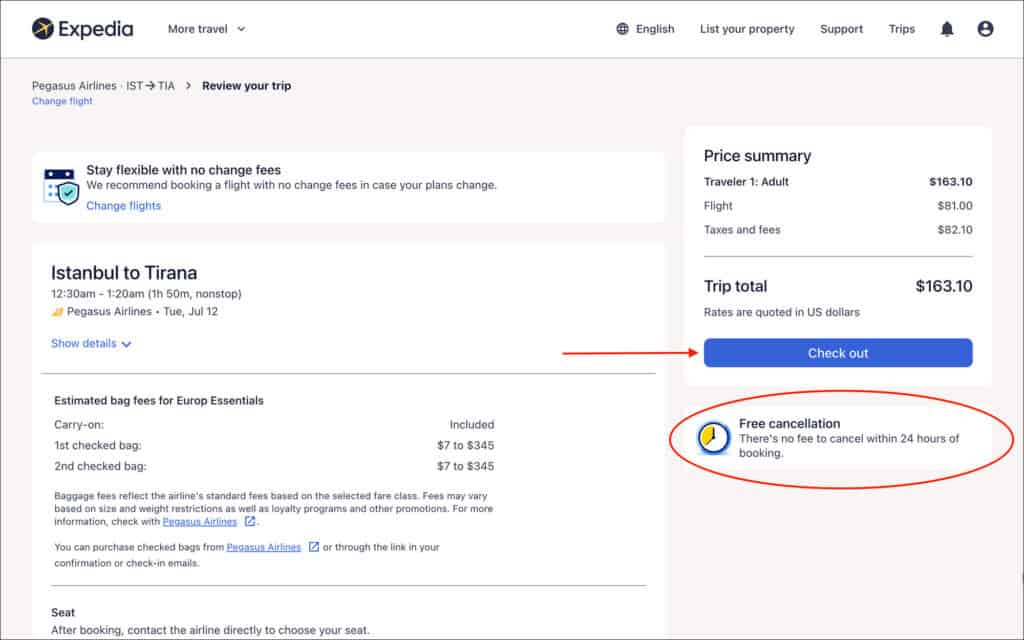Displayed on the screen is an Expedia webpage for booking flights. The webpage features a flight itinerary from Istanbul to Tirana. The price indicated for the journey is $163, though it’s uncertain whether this is for a one-way trip or round trip. Notably, a red arrow points towards a blue "Checkout" button, emphasizing the next step in the booking process. Additionally, a red circle highlights text that reads "Free Cancellation," providing reassurance for flexible travel plans. Interestingly, the breakdown of the total cost shows that the flight itself costs $82, while the combined taxes and fees also amount to $82, highlighting the surprising fact that the ancillary costs are as much as the flight fare itself.